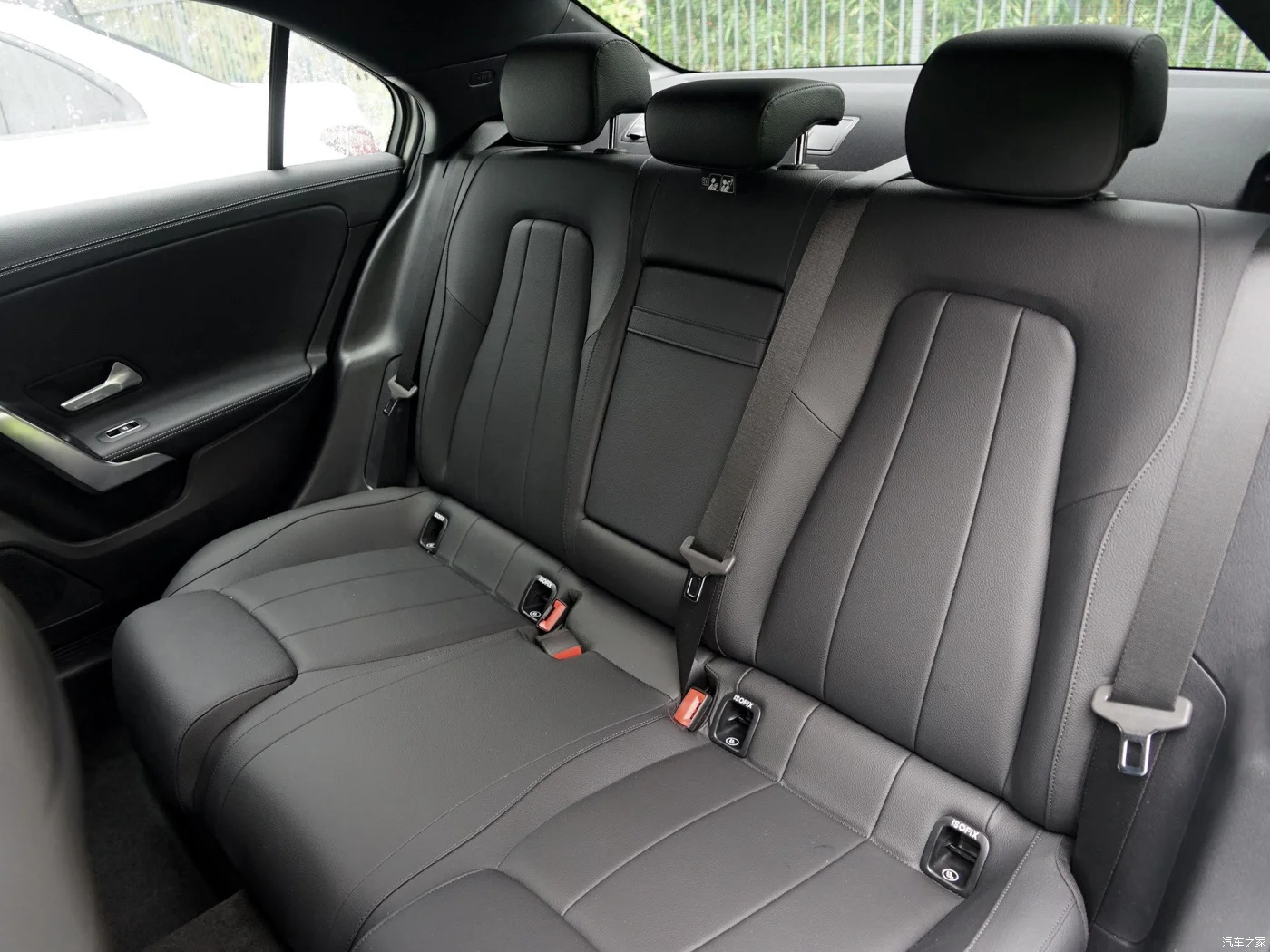The image depicts the interior of a modern car, specifically focusing on the backseat area. The seats are a sleek dark gray fabric and are impeccably clean, suggesting either newness or meticulous upkeep. It is a three-seater arrangement, with all three seats connected and equipped with dark gray headrests; the one in the center is slightly shorter than the others. Each seat is outfitted with a seatbelt, featuring red buckles that are currently not engaged. The car door, visible from the backseat, is a darker gray shade, nearly black, and includes a silver handle. 

The angle of the photograph allows a glimpse into the vehicle’s trunk area, hinting that it might be a hatchback model. Through the car’s rear window, you can spot a fence and some greenery, along with part of a white car parked outside. Additionally, a small portion of the window frame on the top left and a bit of the car’s clean floor can be seen. Overall, the image emphasizes the pristine condition of the vehicle’s backseat, highlighting its modern design and meticulous cleanliness.